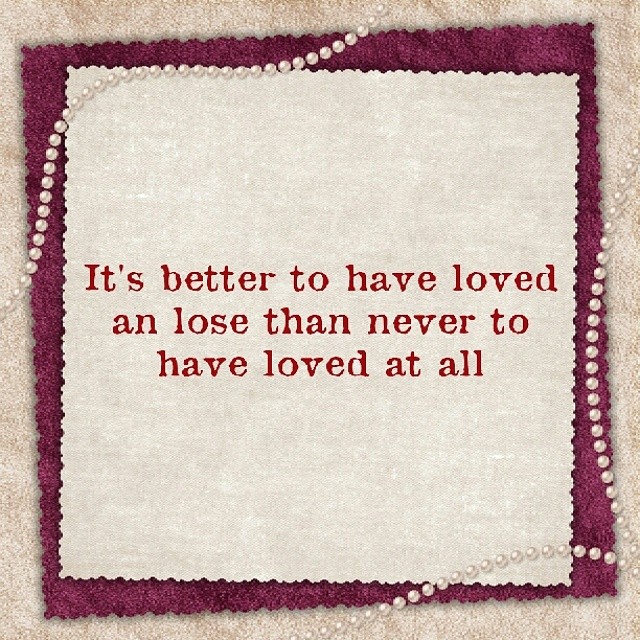This image depicts a visually rich square frame, approximately five inches by five inches, featuring a layered composition. The background consists of a mottled cream and light tan textured surface, creating a sophisticated border. Inside this, a dark mottled fuchsia square positioned slightly askew provides a striking contrast. This fuchsia layer has frilled, slightly ragged edges, contributing to its textured and crafted appearance.

Nested within the fuchsia square is another square with a seemingly uneven placement, resembling white parchment paper, also boasting frilled edges for added texture. Prominently displayed in the center of this parchment layer is a three-line quotation in bold red lettering: "It's better to have loved and lose than never to have loved at all."

The image is further adorned with decorative white pearls. One strand of pearls starts mid-way down the left side, arcing upwards towards the top, while another strand begins at the bottom center, curving to the right and swooping back up. These strands enhance the image's elegant and intricate design, highlighting the central quotation.